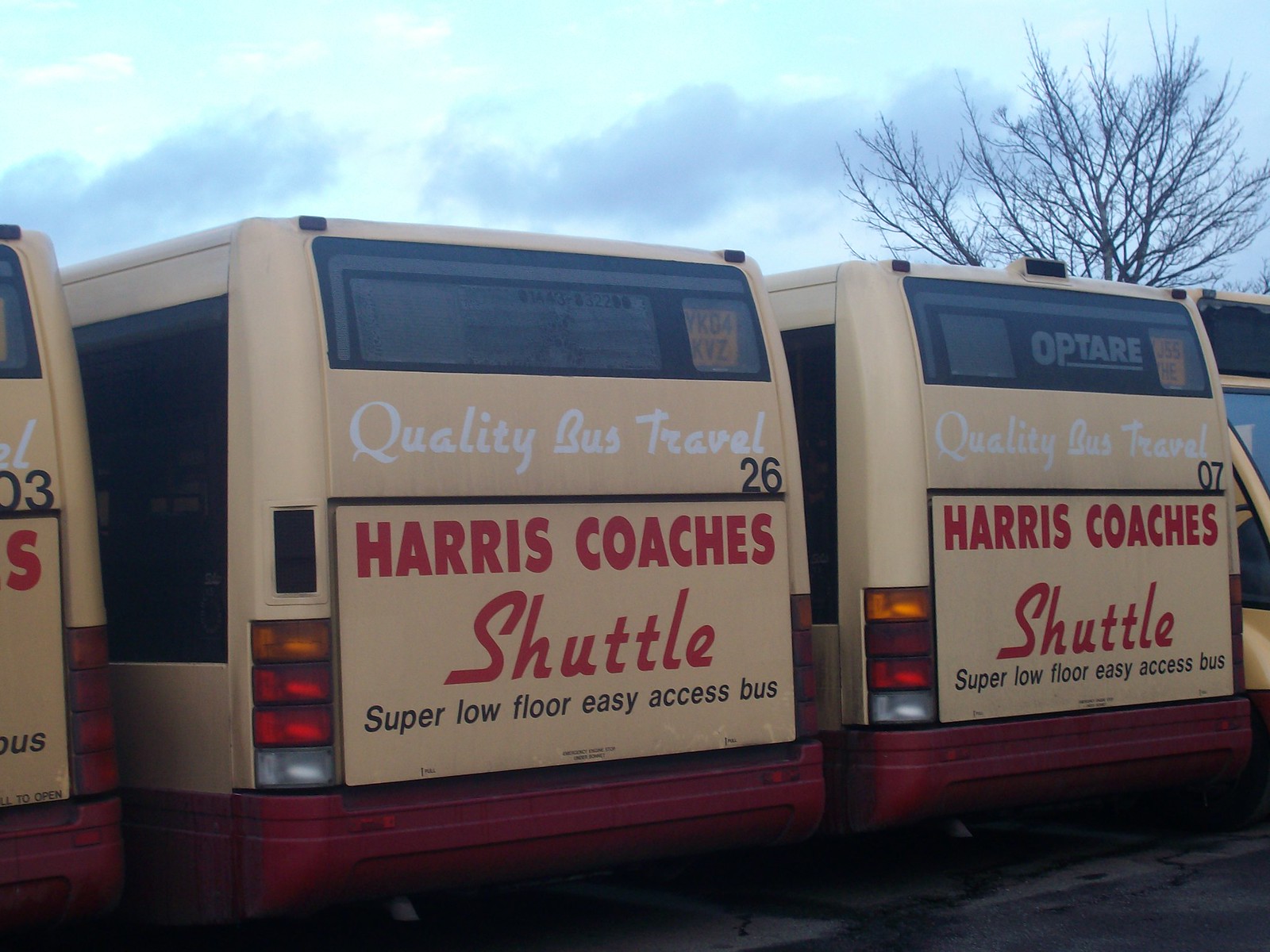This image captures the rear view of three tan-colored Harris Coaches Shuttle buses parked in a lot. The middle bus, prominently displaying bus number 26, features a red bumper and a black "26" on the right side of its back. Above the number, the bus is labeled "Harris Coaches Shuttle" and "Quality Bus Travel" in white text, with the phrases "super low floor, easy access bus" beneath in black. The rear window and a portion of the side windows, which are tinted glass, reveal glimpses of the building situated behind the buses. Similarly, the right bus, numbered 07, follows the same design, with "Quality Bus Travel," "Harris Coaches Shuttle," and "super low floor, easy access bus" labels. A tree with no leaves is visible in the upper right corner of the image. To the far left, a partial view of another bus shows only the "S" from "Harris Coaches" and a portion of the corner. The overall scene suggests a parking lot adjacent to a building, intended for quality coach bus travel services.